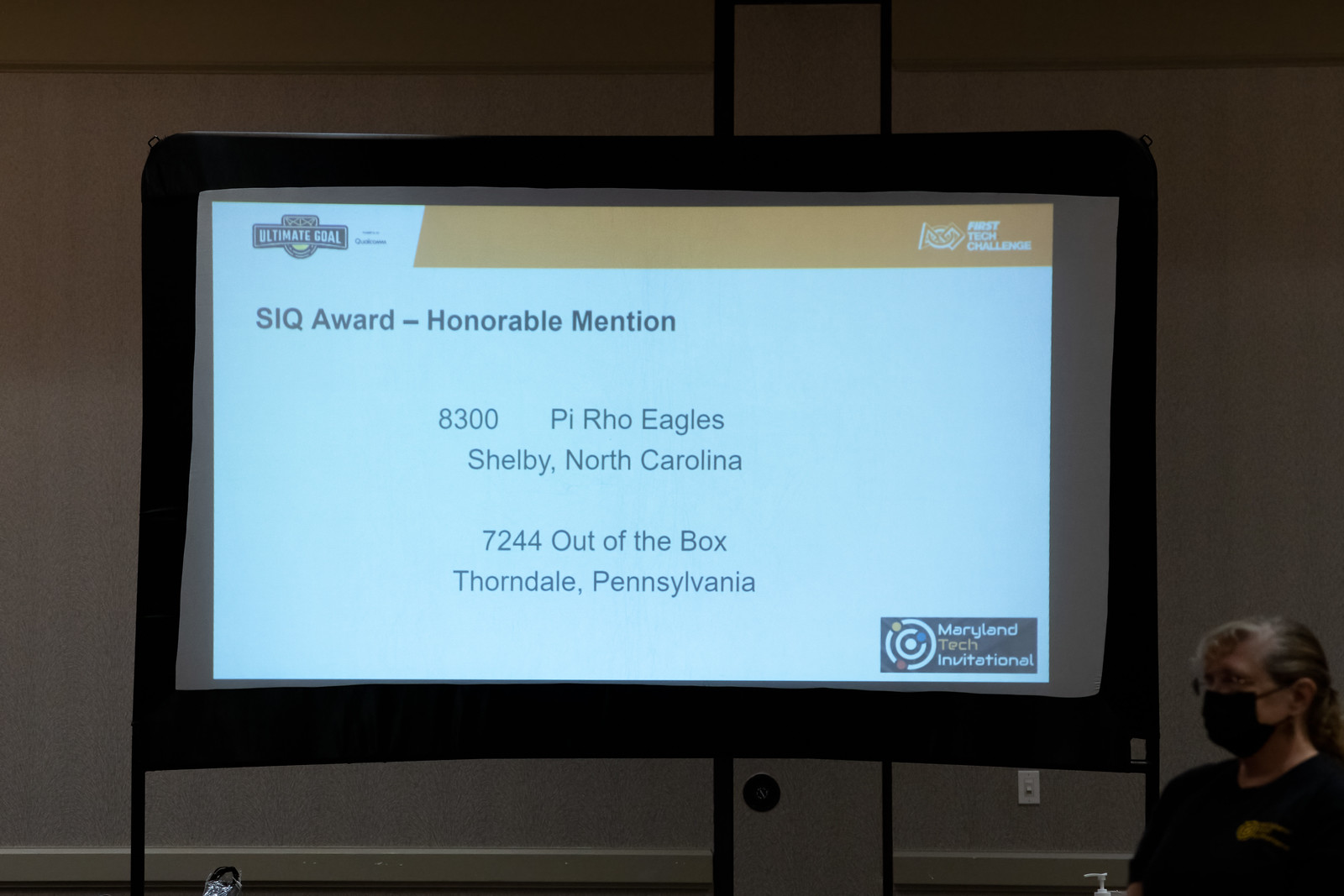The image features a detailed scene set in a conference room, likely within a hotel, characterized by a backdrop or projector screen. The backdrop displays text for a slideshow with the title "Ultimate Goal" prominently positioned at the top left corner. To the top right, within an orange box, the text reads "First Tech Challenge." Below that, in bold black text, "SIQ Award - Honorable Mention" is highlighted. Specific team details are provided, noting "8300 Pyro Eagles, Shelby, North Carolina" and "7244 Out of the Box, Thorndale, Pennsylvania."

In the bottom right corner of the screen, there is a logo resembling a scientific illustration of orbs and atom-like structures, labeled "Maryland Tech Invitational."

To the bottom right of the image, an elderly woman is visible, presumably a participant or attendee. She is wearing a black T-shirt, glasses, and a black face mask, with her gray hair tied back. In front of her is a small bottle of hand sanitizer, indicating preparations for hygiene and safety. The colors of the scene are predominantly gray, gold, black, orange, white, blue, and red, which provide a lively yet professional setting for the presentation.